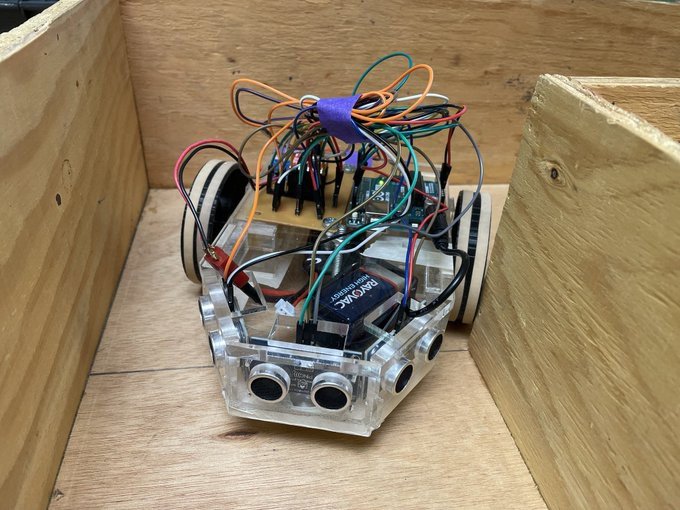This photograph showcases a small, wheeled robot navigating through a maze constructed from light-colored plywood. The rectangular picture reveals a detailed view of the robot facing towards the user, situated amidst the maze's 90-degree angled wooden walls, which are slightly taller than the robot itself. The robot features a clear plastic body with a predominantly rectangular bottom half and a hexagonal top half. It is intricately connected with an array of exposed wires—green, orange, red, white, and black—linked to a motherboard located towards the rear of the device. The electronics include a prominent Rayovac battery situated in the front left section, alongside various sensors. Six black felt circles, resembling eyes, encircle the robot's base, two in the front and two on each side. The two wheels are positioned at the rear, propelling the robot through the maze, which appears to be about a foot in height. The clear, plastic platform constitutes the base, while a dual-layer assembly is evident, with some components mounted on top and others beneath the panels. The detailed wiring is neatly fastened by a thick purple ribbon, providing a complex yet organized appearance to the sophisticated miniature robot vehicle as it maneuvers through the wooden labyrinth.